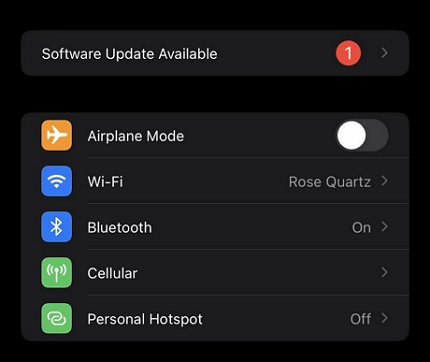The image depicts a section of a cell phone screen with a predominantly black background and various interface elements slightly differing in shade. At the top, there is a notification in white text stating "Software update available," accompanied by a red square containing the number '1' in white. Below this notification, there are five distinct rows, each featuring an icon and text indicating different settings.

1. **Airplane Mode**: The first row has an orange square with a white airplane icon. To its right, the text "Airplane Mode" is displayed in white, alongside a toggle switch icon that is positioned to the left, with a white circle indicating the current inactive state.
   
2. **Wi-Fi**: The second row showcases a blue square with the Wi-Fi symbol. Adjacent to it, the label "Wi-Fi" appears in white text, followed by the network name "Rose Quartz" on the same line.
   
3. **Bluetooth**: The third row includes a blue square containing the Bluetooth symbol. The accompanying text "Bluetooth" is in white, and to the right, it states "On," indicating that Bluetooth is currently enabled.
   
4. **Cellular**: The fourth row features a green square with a cell signal icon. The text "Cellular" is positioned next to the icon, with a right-facing caret symbol to the right, but no additional text is provided.
   
5. **Personal Hotspot**: The fifth row displays a square with white interlocking rings, symbolizing a personal hotspot. The label "Personal Hotspot" is in white text, accompanied by the word "Off" and a right-facing caret indicating that the hotspot is not active.

This portion of the cell phone screen effectively illustrates the status of various settings and highlights the availability of a software update.